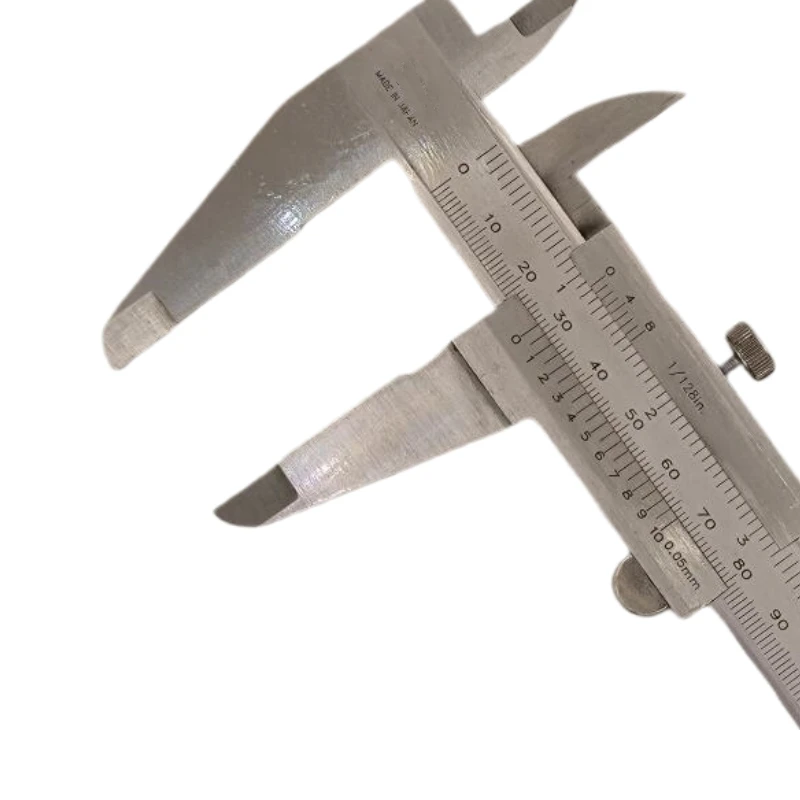The image features a detailed close-up of a Vernier caliper against a stark white background. The caliper is a precise measuring instrument, depicted in a monochromatic gray color. The image is cropped, showing only the upper portion and cutting off the lower right section of the tool. The caliper consists of a main scale marked with clear, ascending increments (0, 10, 20, 30, 40, 50, 60, 70, 80, 90), and a sliding vernier scale for finer measurements, possibly in millimeters. Two prominent jaws are found on the left, resembling the open mouth of a creature such as a Tyrannosaurus Rex, used for measuring the external dimensions of objects. On the opposite end, smaller inner jaws and a calibration knob are visible, enhancing its functionality. The caliper also has "Made in Japan" inscribed in black, indicating its origin. The tool extends diagonally across the frame from the upper left to the lower right, emphasizing its elegant and precise design.